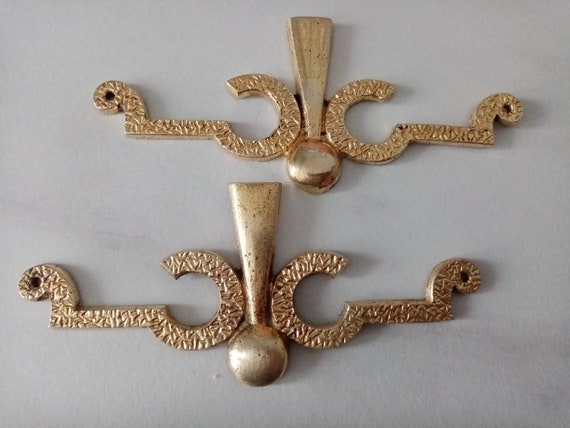This image showcases two identical wall decorations set against a white background, one positioned slightly below and to the left of the other. Both decorations prominently feature a central element resembling an exclamation point in a gold chrome or pale bronze color. This central exclamation mark is flanked on each side by mirror-imaged components that start as a "C" or reverse "C," extending horizontally before curving upwards into a small circle with a hole in the center, evoking the appearance of a small snake. The ornaments are characterized by numerous small indentations resembling carved random lines along the curved and horizontal segments. Despite their slight thickness, they seem to serve solely as decorative pieces with no apparent functional use beyond aesthetic appeal. The decorations exhibit a slightly worn look, with one appearing in marginally better condition than the other.